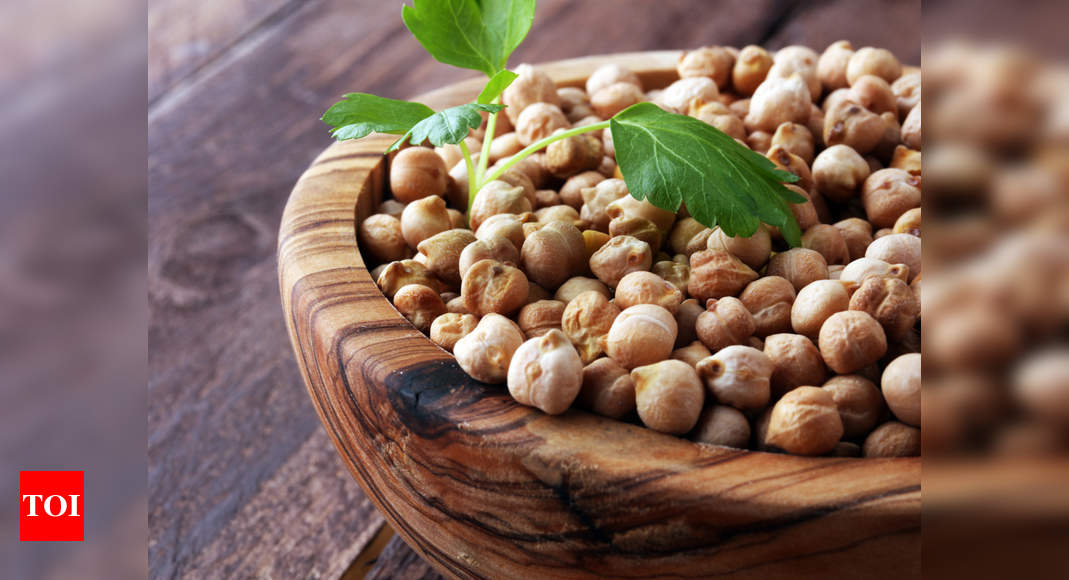In this photograph, we see a hand-carved wooden bowl brimming with numerous round, light brown nuts, possibly macadamia or hazelnuts, each with a slight white shading. The bowl is adorned with a sprig of greenery, perhaps mint or parsley, adding a contrasting touch of green to the overall brown ensemble. The bowl itself rests on a rustic wooden surface, likely a picnic table or hardwood floor, featuring visible dark wood grain that enhances the natural and earthy ambiance. The background incorporates varying shades of lavender, purple, and black, adding a soft, artistic touch. To the bottom left of the image is a red square with the white letters "T-O-I," possibly indicating a brand name. Notably, the right side of the bowl and some of its contents appear slightly blurred, adding an intriguing visual element to the composition.